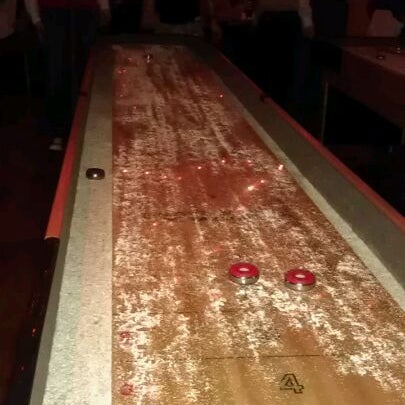The image depicts a dark room centered around a worn-out tabletop shuffleboard. The shuffleboard, made of scraped and weathered light-colored wood with tan and gray borders, extends back into the darkness of the room. Mid-image, two red-topped, metallic markers and a single silver one are visible; the red markers have white circles with visible dots above the midline. Positioned near the number four, these markers highlight the game's active play area. The shuffleboard stands out starkly against the dim surroundings, drawing attention to its aged condition and the action happening on its surface.